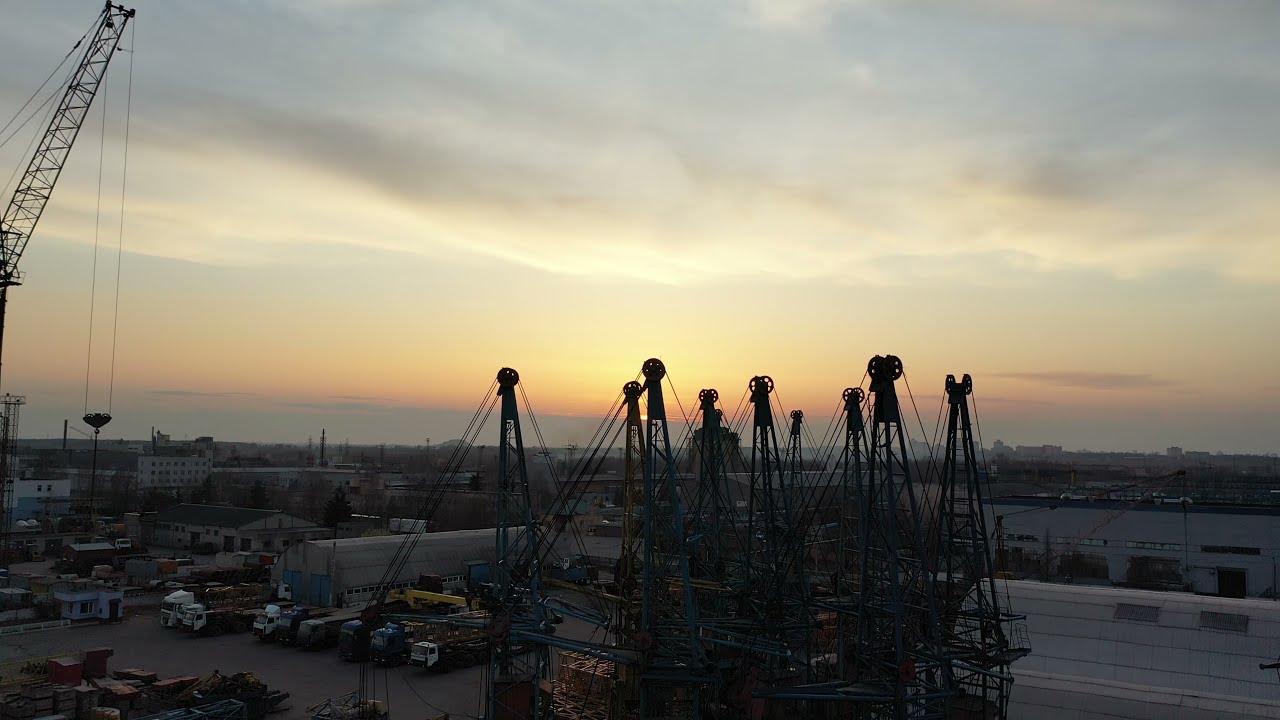The image showcases a high-angle, aerial view of an industrial yard, likely a shipyard or a crane storage facility, situated next to a river in an urban area with a city skyline in the background. At dusk, the scene is bathed in a warm, golden-orange hue from the setting sun, and some structures are backlit, casting detailed silhouettes. Central to the image is a collection of cranes, approximately ten in total, painted in blue and yellow, folded and bunched together. There is a larger crane to the left, extended upwards, along with an array of construction and hauling vehicles beneath, including flatbed trucks, semi-trailers, and a dump truck. On the bottom right, there are large warehouse buildings and storage areas, further suggesting industrial activity. The scene hints at an organized operational yard with a variety of machinery and vehicles, aligning with either shipbuilding or heavy-duty construction work.